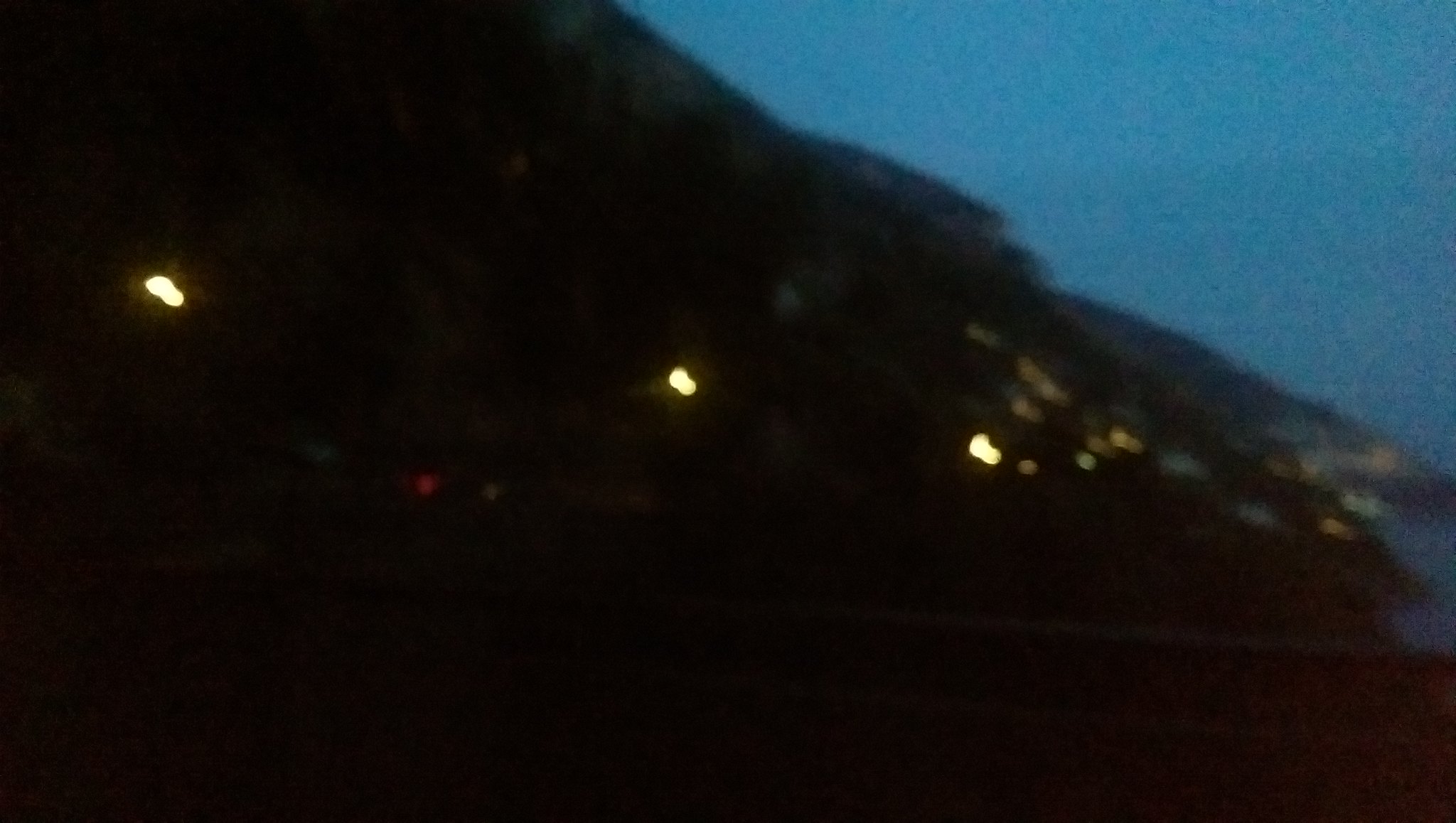This photograph appears to capture a dimly lit and blurry nighttime scene of a coastal landscape, potentially seen from a drone or an elevated perspective. The image features a dark, winding road illuminated by three distinct street lights, which guide the viewer's eye towards a small town or harbor area near the coast. To the right, there's a patch of deep blue sky or ocean, creating a subtle contrast against the surrounding darkness. A faint red light, possibly the backlight of a car, is visible on the road. The scene is slightly tilted, adding to the disorienting and fuzzy quality of the image, but the coastal cliffs, street lights, and the hint of a distant town make it a distinctive and intriguing landscape.